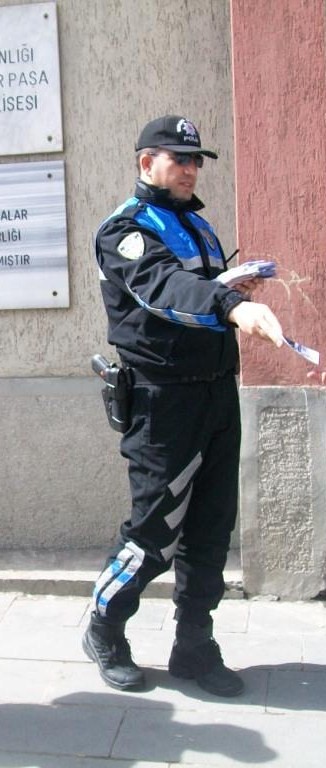The photograph captures a Caucasian police officer, estimated to be in his 30s or 40s, standing outside on a sunny day, likely on a cement or tiled sidewalk. He is wearing a dark baseball cap adorned with white text resembling "police" or its translation in another language. His attire includes a black and medium blue windbreaker-style jacket, complete with a black collar zipped to the top, and dark sunglasses shielding his eyes. The jacket bears on one shoulder and the front breast, logos or emblems signifying his authority. He is equipped with a gun in a holster on his right hip, black pants featuring some white rectangular designs on the lower right leg, and black boots. In his left hand, he holds a stack of pamphlets or a notebook, while his right arm extends forward, offering one document to an unseen person outside the frame. His shadow is cast in front of him alongside the shadow of another unseen individual. The backdrop includes a combination of gray and reddish brick or concrete wall, possibly the side of a historical or religious building, with partially visible marble signs etched in black. One sign appears to include the Spanish word "PASA" further suggesting an international setting.